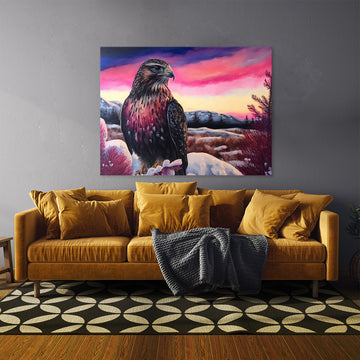This image features a cozy living room with a wooden floor and a distinctive black and white geometric area rug, characterized by a pattern of ovals and circles forming a near-diamond design. Dominating the scene is a luxurious gold-colored velvet couch, supported by four wooden legs. The couch is adorned with seven fluffy cushions—arranged with two on each end and three along the center—and a blue throw blanket draped invitingly across its seat, hinting that someone recently rested there. Above the sofa hangs an elaborate painting of a gray and pink bird, possibly a falcon or hawk, perched on rocks. The bird is thoughtfully gazing to the right, framed by a picturesque landscape with a gradient sky transitioning from bluish-purple at the top to pink, white, and yellow near the horizon. The backdrop also includes distant mountains and a hint of pine trees, adding depth and serenity to the scene. The picture, alongside the soft, plush furniture, creates an inviting and cozy atmosphere in the room.